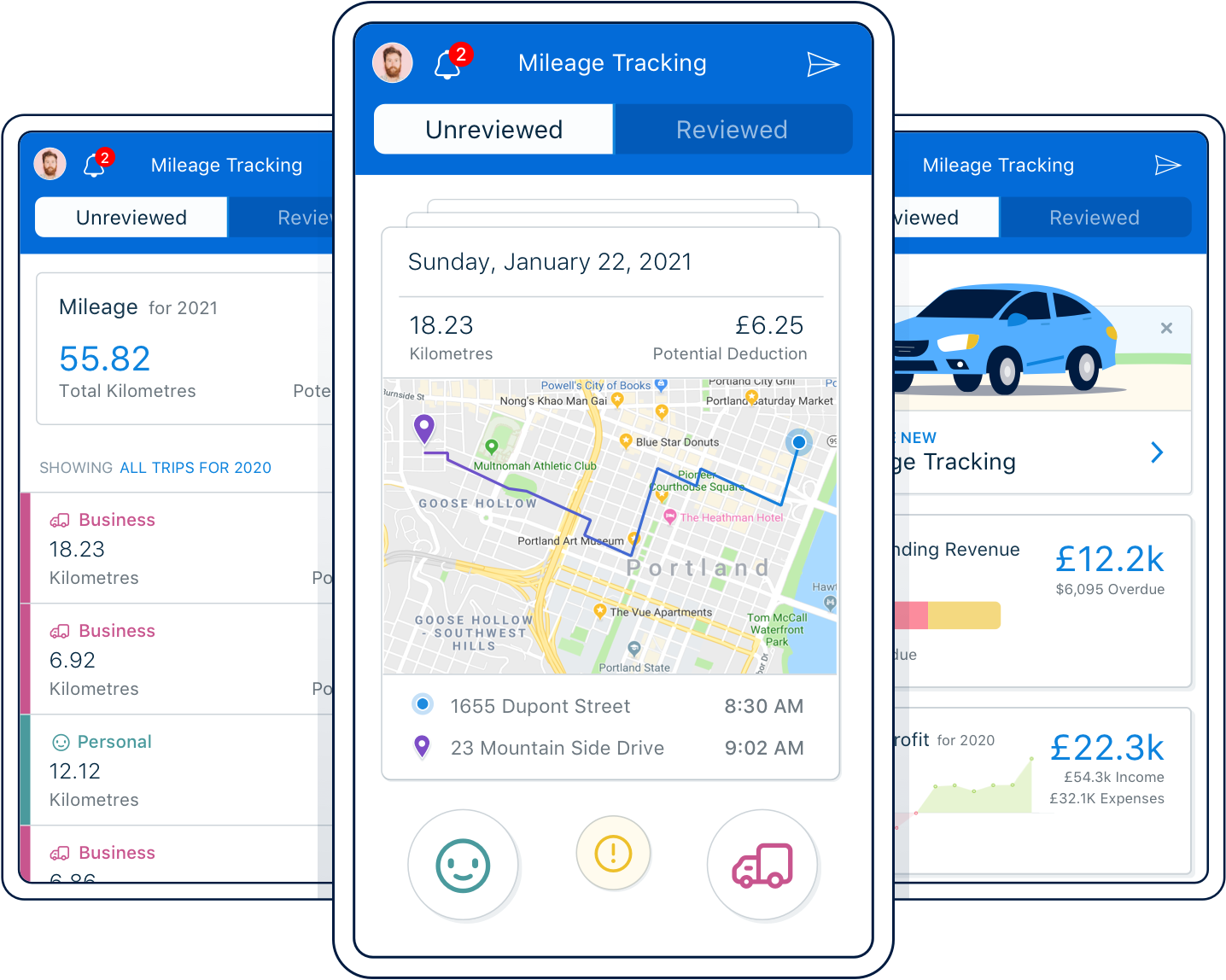This detailed infographic visually presents a mileage tracking application across three smartphone mockups. 

In the background, two smartphones are angled to the left and right. The central smartphone prominently overlaps these, ensuring focus. All three screens display the "Mileage Tracking" feature underlined in white text.

Each device screen is set to the "Unreviewed" tab, which is one of the two tabs available along with "Reviewed." The leftmost smartphone showcases "Mileage for 2021" with numerical data highlighted in blue. Beneath this, it lists trips under the heading "Showing all trips for 2020."

The central smartphone features a carousel of trip details, the foremost being a trip from Sunday, January 22, 2021. This trip records 18.23 kilometers traveled, potentially deducting £6.25. A large map dominates the lower section, pinpointing start and end locations. At the bottom, it lists the specific addresses of departure and arrival, along with their respective times. Three distinct emojis appear at the bottom: a green smiley face, a yellow exclamation point, and a purple box truck icon.

The rightmost smartphone features an image of a car at the top, paired with the "Mileage Tracking" heading below. The right side of this screen displays two amounts within white boxes, contributing to the detailed breakdown of the application's mileage tracking capabilities.